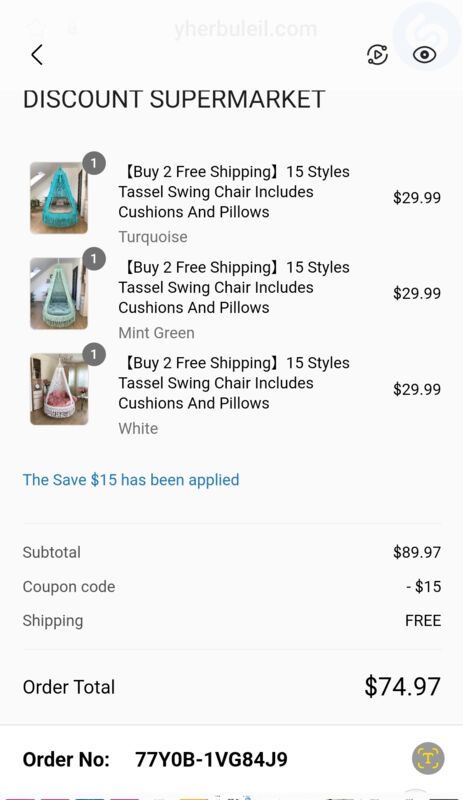Here is a detailed and cleaned-up caption for the image:

"This image captures a smartphone screen displaying a shopping page from 'Discount Supermarket.' At the top, a black arrow points left, followed by the store's name in bold capital letters. Below that are three product listings for chairs, each enclosed in its own rectangular box. Each box has a gray circle at the top-right corner, slightly overlapping, with the number "1" inside, written in white.

The first product is a tassel swing chair in turquoise, described as 'buy two, free shipping,' and offering 15 styles. It includes cushions and pillows and is priced at $29.99. The subsequent two products are identical chairs in different colors: mint green and white, both priced at $29.99.

Below these listings, a message in blue text reads, 'Save $15 has been applied.' Further down, the subtotal, coupon code, and shipping details are filled out. The page also includes an order number prominently displayed in bold black ink."